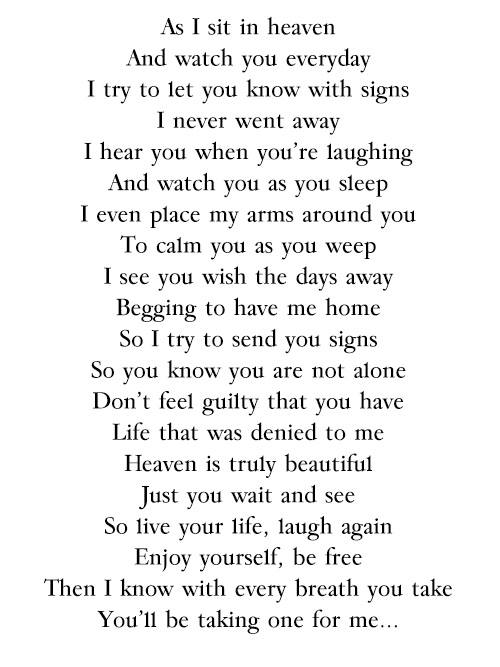The image depicts a simple yet poignant black text on a white background. The text is arranged vertically in a common, easy-to-read font. It delivers an emotional message from a loved one who has passed away, speaking directly to those left behind. The quote reads: "As I sit in heaven and watch you every day, I try to let you know with signs I never went away. I hear you when you're laughing and watch you as you sleep. I even place my arms around you to calm you as you weep. I see you wish the days away, begging to have me home, so I try to send you signs so you know you are not alone. Don't feel guilty that you have life that was denied to me. Heaven is truly beautiful, just you wait and see. So live your life, laugh again, enjoy yourself, be free. Then I know with every breath you take, you'll be taking one for me." This deeply touching message captures the essence of eternal love and the enduring presence of those who have passed, offering comfort to the grieving by assuring them of continual, unseen support from above.